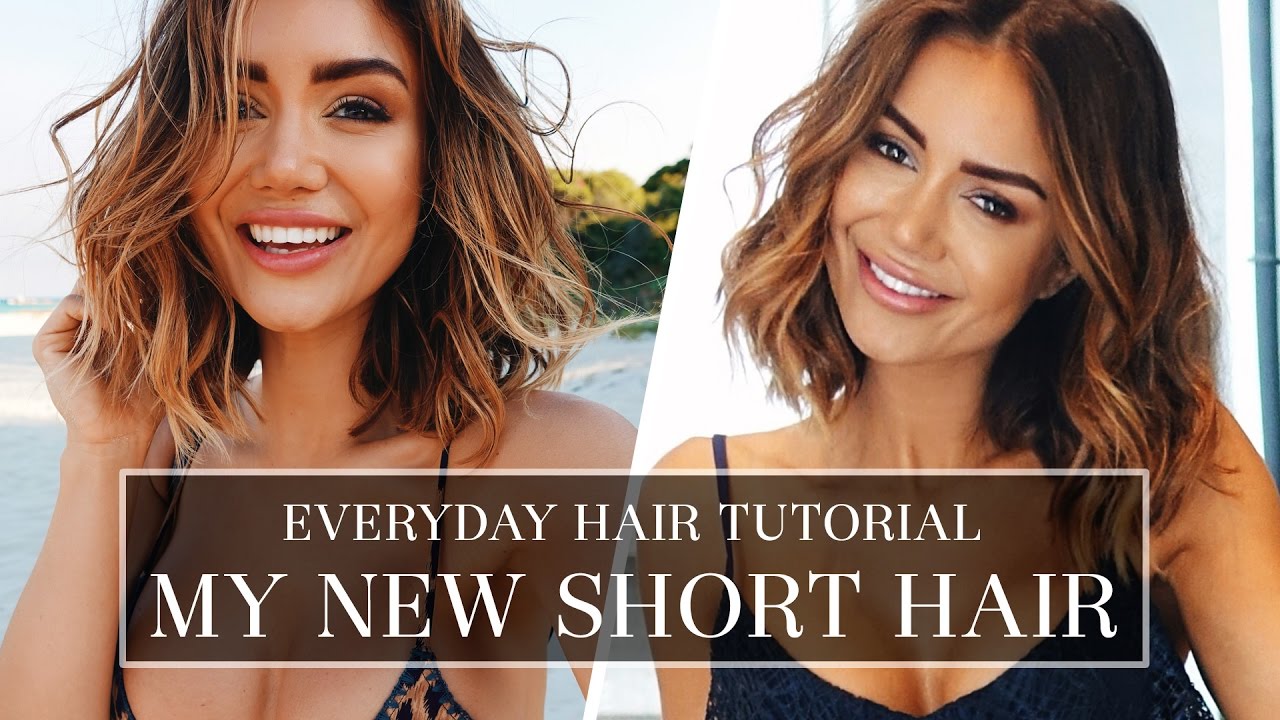The image consists of two frames side-by-side. Both frames appear to feature a single woman in two different settings. In the left frame, the woman is outdoors, likely at a beach, evidenced by the visible ocean and trees in the background. She has short, dark brown hair with hints of light brown highlights, styled in a curvy manner. She is smiling brightly with her teeth visible, wearing makeup that includes lipstick and eye makeup, and sporting a sun dress. Her hand is gently touching her hair, adding to her cheerful and relaxed demeanor.

In the right frame, the same woman is indoors, maintaining the same hairstyle and makeup. She continues to smile, showcasing her lively spirit. She is dressed in a blue-colored sun dress, standing against a well-lit background that enhances the clarity and brightness of the image.

Across both frames, there is a transparent brown text box with white capitalized letters that reads "Everyday Hair Tutorial, My New Short Hair." The text underscores the thematic focus on showcasing her new hairstyle. The overall image is vivid and well-lit, making the details of her appearance and surroundings easily discernible.